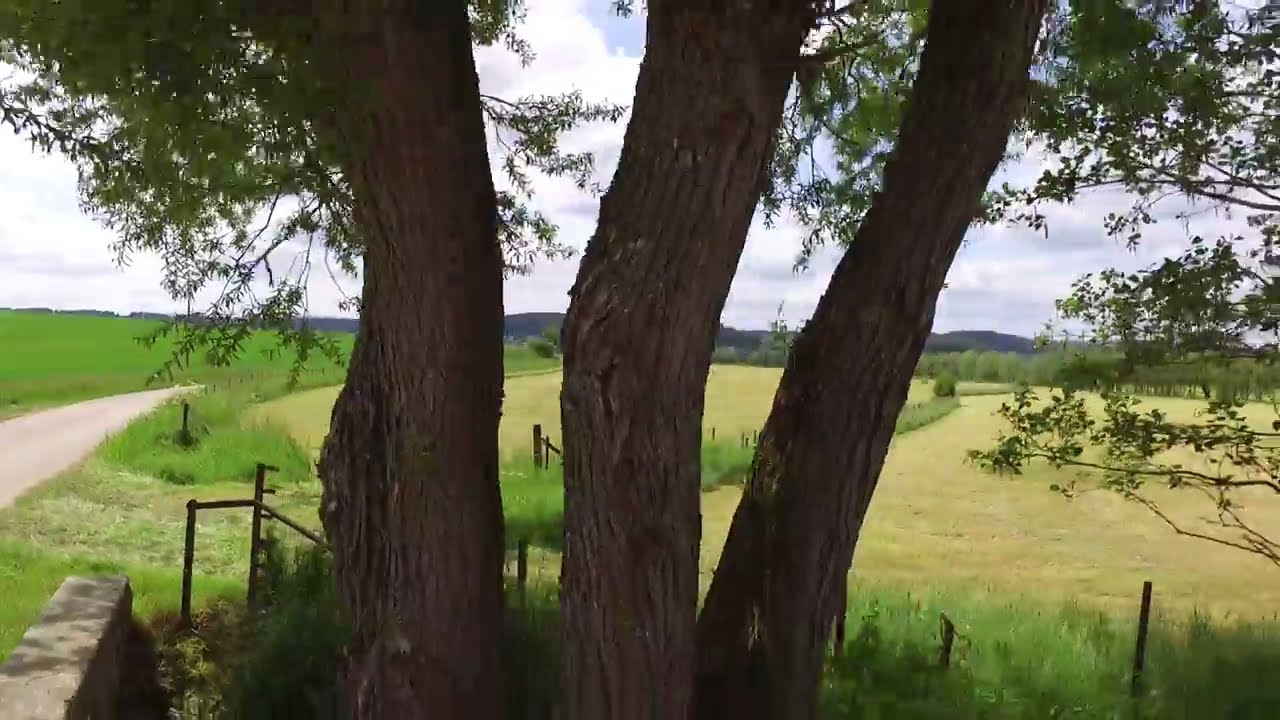In the foreground of the image, three tree trunks, possibly belonging to separate trees, stand close together. The trunks are not entirely straight, and their branches, situated high up, are adorned with small green leaves. You can see the scattering of some leaves around the trunks. The setting is partly sunny, casting faint shadows around the trees and highlighting the vibrancy of the scene.

Behind these trees, an expansive, largely empty field stretches out, characterized by green grass and a few patches of taller grass. Some metal fence posts are visible behind the trees, though the fence wiring is too faint to be seen clearly. On the left side of the field, a gravel road cuts through the grassy expanse, leading towards the horizon. 

In the distance, a faint line of hills marks the horizon under a bright blue sky dotted with white clouds. The field seems to be split by a fence in the middle-ground, creating a green space that delineates two separate sections of the field. Overall, the scene captures a serene, rural landscape under a sunny sky.